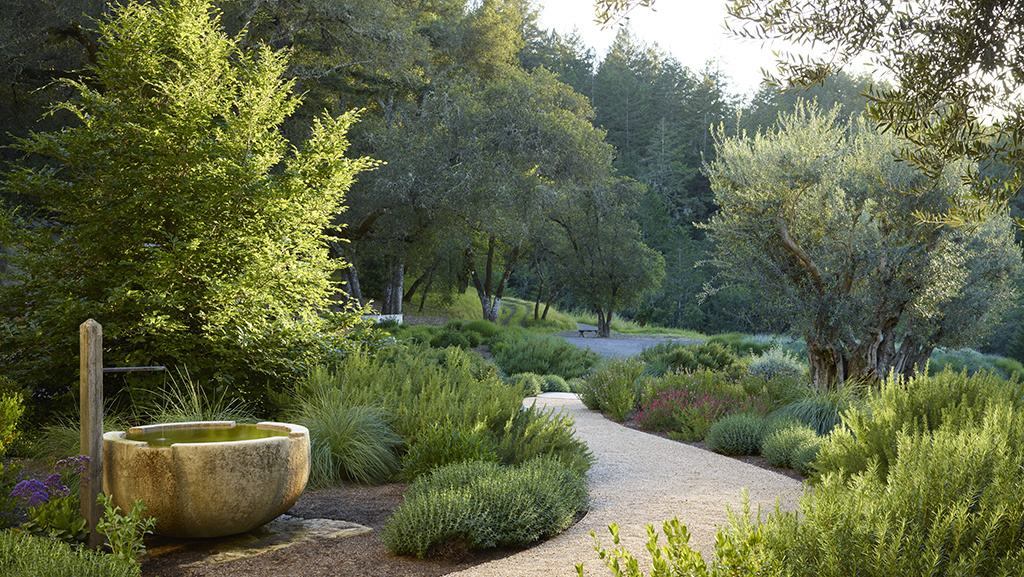This color photograph captures a serene garden scene bathed in daylight. The center of the image is dominated by a meandering walkway made of light brown stone or gravel, which begins at the bottom center and curves leftward before winding back around through the lush greenery. Tall, verdant trees cluster together in the background, their tops framing a clear blue sky. Closer to the camera, various shades of green shrubbery and small trees dot the landscape.

On the left near the start of the walkway, a distinctive water fountain can be seen—a large, bowl-shaped stone structure with a wooden post and a pipe dripping water, surrounded by purple flowers. Next to it is a small tree. Further along the path, a section filled with blue flowers appears, adding splashes of color to the scene. A park bench is situated in the distance on a gray gravel area, offering a place to rest and enjoy the tranquil setting. Another connected pathway ascends a grassy hill in the background, flanked by more trees. This detailed and vibrant image encapsulates the peaceful harmony of nature and thoughtful garden design.